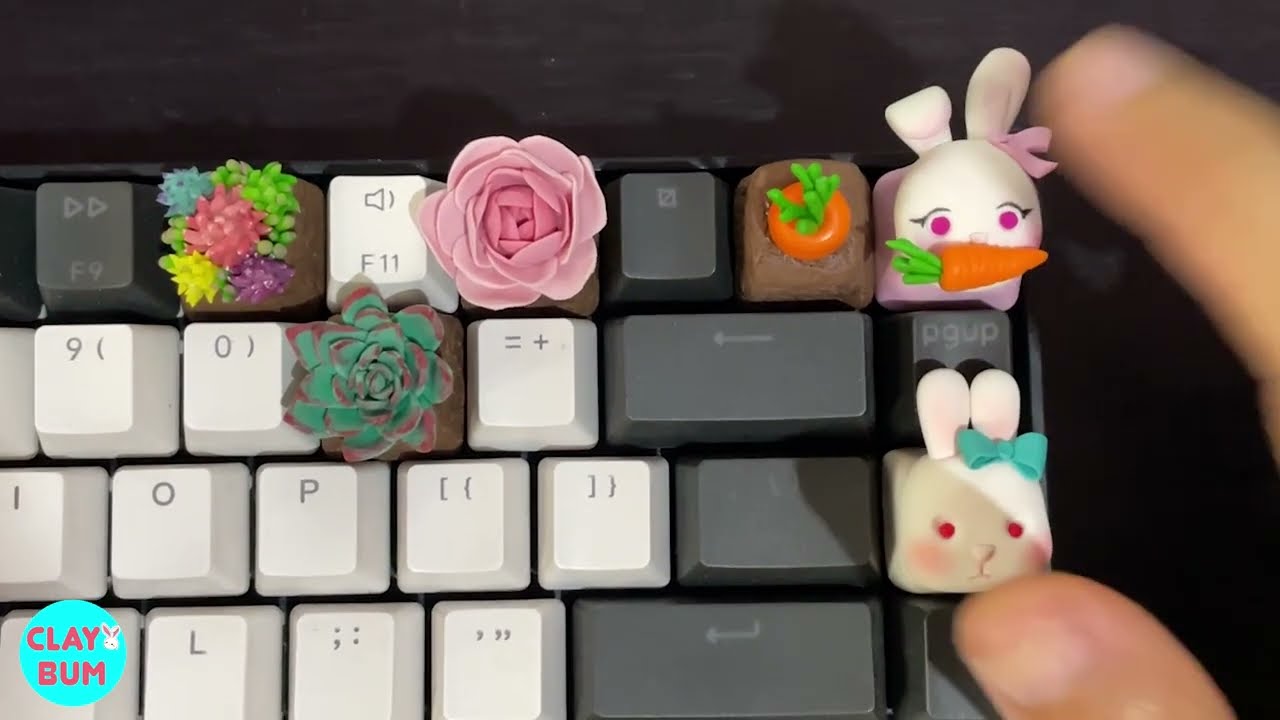This close-up photograph features the top right portion of a full-size computer keyboard, viewed from above. The keyboard keys are black and white, spanning from F9 on the top row to the Delete key on the far right, with the bottom row visible starting from L to the right. Several keys are adorned with customized clay decorations: a brown flowery clay piece covers the F10 key, a clay rose adorns the F12 key, and a leafy design decorates the dash key next to the zero. On the top right, one key has a brown base with an orange carrot, while the adjacent key showcases a white rabbit holding a carrot in its mouth. Two rows below, another white rabbit with a blue bow is present. Visible in the image are two fingers, with a thumb near the blue bowed bunny and an index finger near the bunny with a carrot. The background appears to be a black desk with paint gaps. In the bottom left corner, a small blue circle features the brand name "Clay Bum" in pink text.